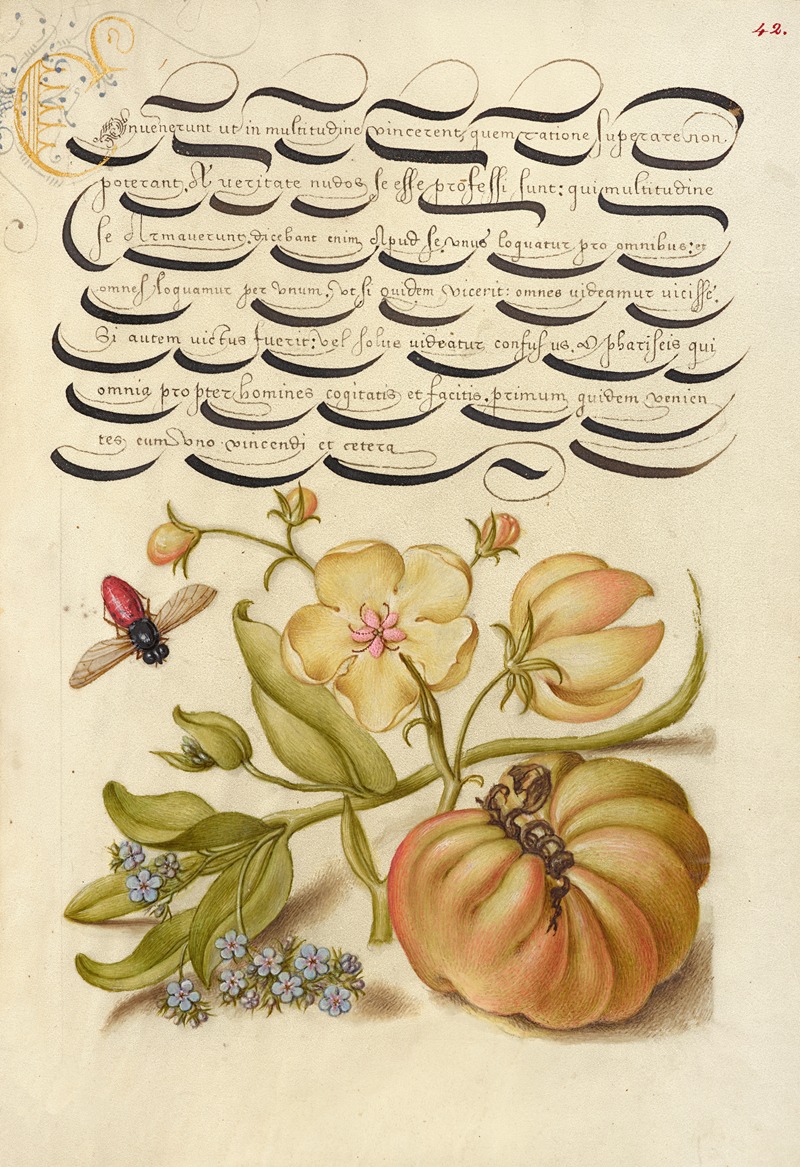This poster is an intricately detailed drawing on a beige, aged, and slightly browned background, hinting at its old age. At the top, the page is numbered 42 in red ink. Dominating the upper section is a highly stylized, ornate script reminiscent of Middle Eastern calligraphy, featuring thick black swirls and intricate little scripts now somewhat faded. In the upper left corner, a small gold symbol catches the eye.

The bottom part of the poster features a detailed biological illustration. Central to the composition is a winged insect with a red body. Surrounding the insect are various flowers, including small blue forget-me-nots and larger, faded yellow flowers with pink centers. Among the flora, a fruit resembling a pomegranate sits with a coiled vine around it, bearing reddish tones. This vine and fruit add a layer of complexity to the botanical array. The harmonious blend of text and imagery provides a rich visual experience, evoking both natural beauty and linguistic artistry.